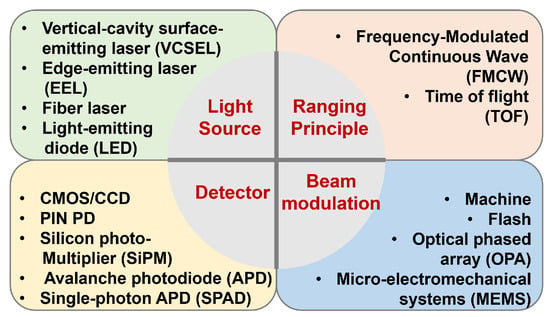The image appears to be an educational diagram from a scientific journal or textbook, featuring four distinct yet interconnected colored sections, each annotated with detailed information about different components related to a system involving light and detection principles. 

In the top left, within a light green square labeled "Light Source," it lists various types of emitters, including vertical cavity surface emitting lasers (V-C-S-E-L), edge emitting lasers (E-E-L), fiber lasers, and light emitting diodes (L-E-D). The top right section, in light red, is labeled "Ranging Principle" and includes frequency modulated continuous wave (F-M-C-W) and time of flight (T-O-F) techniques. The bottom left, colored light yellow, is marked "Detector" and details sensors such as CMOS (Complementary Metal-Oxide-Semiconductor), CCD (Charge-Coupled Device), pin photodiode (P-D), silicon photomultiplier (SiPM), avalanche photodiode (A-P-D), and single photon avalanche diode (S-PAD). Finally, the bottom right, in light blue, is labeled "Beam Modulation," encompassing technologies like machine flash, optical phased array (O-P-A), and microelectromechanical systems (M-E-M-S).

At the center of these four quadrants is a gray Venn diagram-like circle, divided into four sections, each corresponding to one of the labeled squares, with the respective categories written in red text within their segments of the circle.